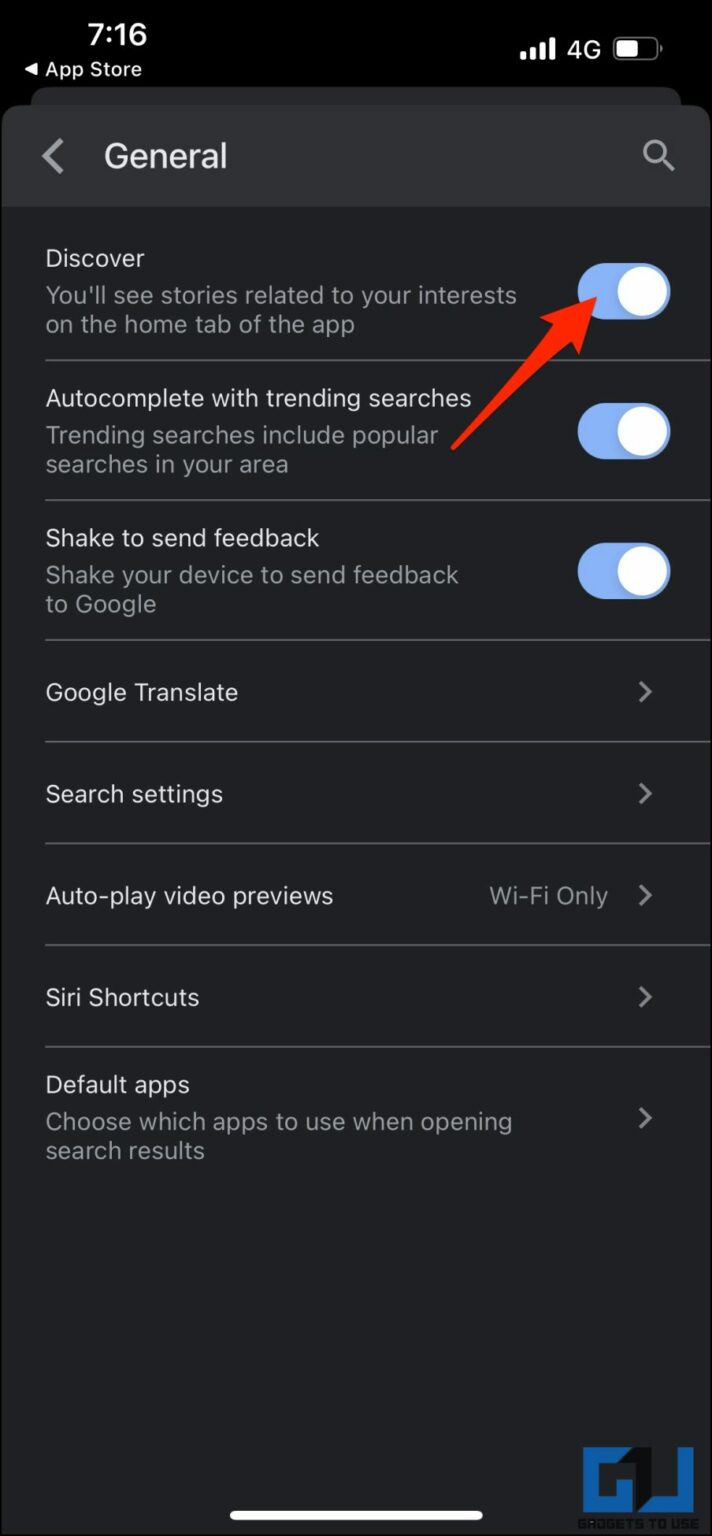The image captures a screenshot from a mobile phone displaying the general settings of an app. In the upper left corner, the time is shown as 7:16. On the upper right, the signal strength icon displays full bars, indicating a strong 4G connection. Adjacent to this is the battery icon, which is approximately 60-70% charged.

Below the status icons, the word "General" is prominently displayed, followed by a search bar on the right side of the screen. Detailed settings beneath include:

1. **Discover**: "You'll see stories related to your interests on the home tab of the app."
2. **Autocomplete with Trending Searches**: "Trending searches include popular searches in your area."
3. **Shake to Send Feedback**: "Shake your device to send feedback to Google."
4. **Google Translate**: This option appears next in the list.
5. **Search Settings**: This is another available setting.
6. **Autoplay Video Previews**: With the status "WiFi only" activated.
7. **Siri Shortcuts**: Listed as another setting.
8. **Default Apps**: "Choose which apps to use when opening search results."

The entire screenshot maintains a clean, rectangular shape.